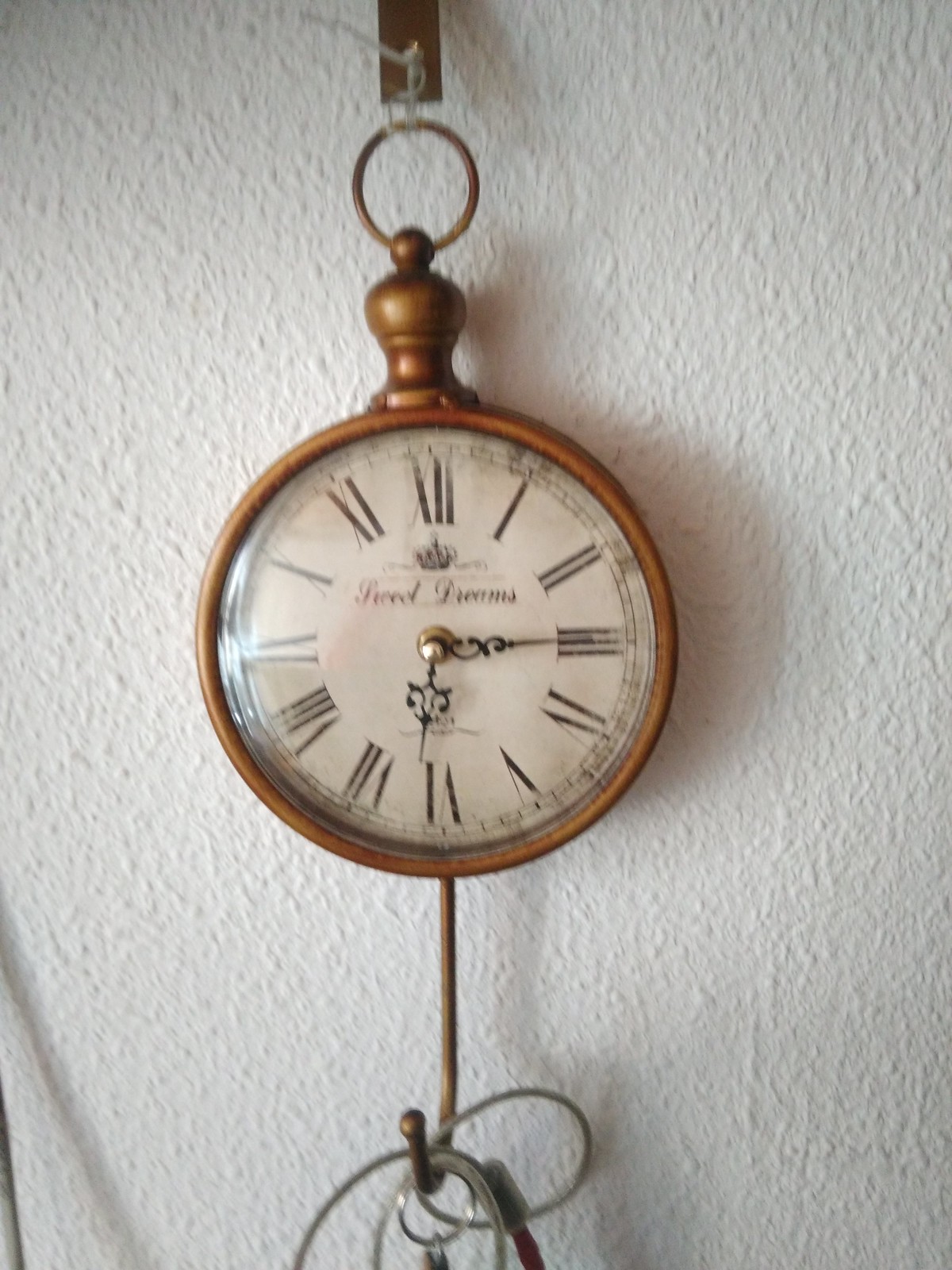A photograph captures a vintage wall-mounted watch prominently displayed against a stark white, painted wall. The timepiece features a sophisticated brown frame, contrasting elegantly with its white face. The watch's center, where the hands—black and slender—point at Roman numeral hour markers, creates a focal point of timeless elegance. Suspended from a hook at the top, the watch also has a decorative brown element near its upper edge and a small brown ring securing it to the hook. Below the watch, another larger hook holds several gray rings, possibly keys, adding a utilitarian touch to the scene. The composition centers the watch on the white wall, making it the unmistakable highlight of the photograph. No other objects or distractions are present, ensuring the viewer's attention remains solely on the ornate timepiece and its immediate surroundings.